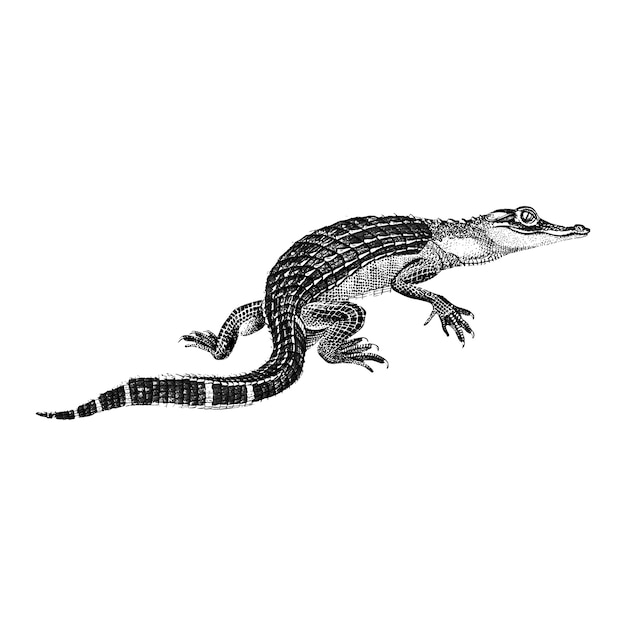The image is a detailed black and white line art illustration of a caiman alligator set against a plain white background, giving it a floating appearance. The caiman, rendered with fine pen or pencil-like precision, is depicted in profile, facing the right-hand side of the image. Its body extends from the middle of the picture towards the lower left corner, where its tail curves and tapers. The caiman's pointed head features large, round, and bulbous eyes that seem to look directly at the viewer. The snout is short and thin with raised nostrils, while the mouth, closed, is accentuated with a long line extending past the eye. The neck is notably bulbous and flares into the shoulders, which give way to a back adorned with dark, raised scales that contrast with the lighter-colored neck. These scales continue down its length, forming a distinctive white stripe effect. The short, bent limbs are equipped with five clawed fingers and toes, adding to the creature's reptilian intricacy. The overall length of the caiman is approximately four inches, with the potential to appear longer if not for the curvature of its tail.